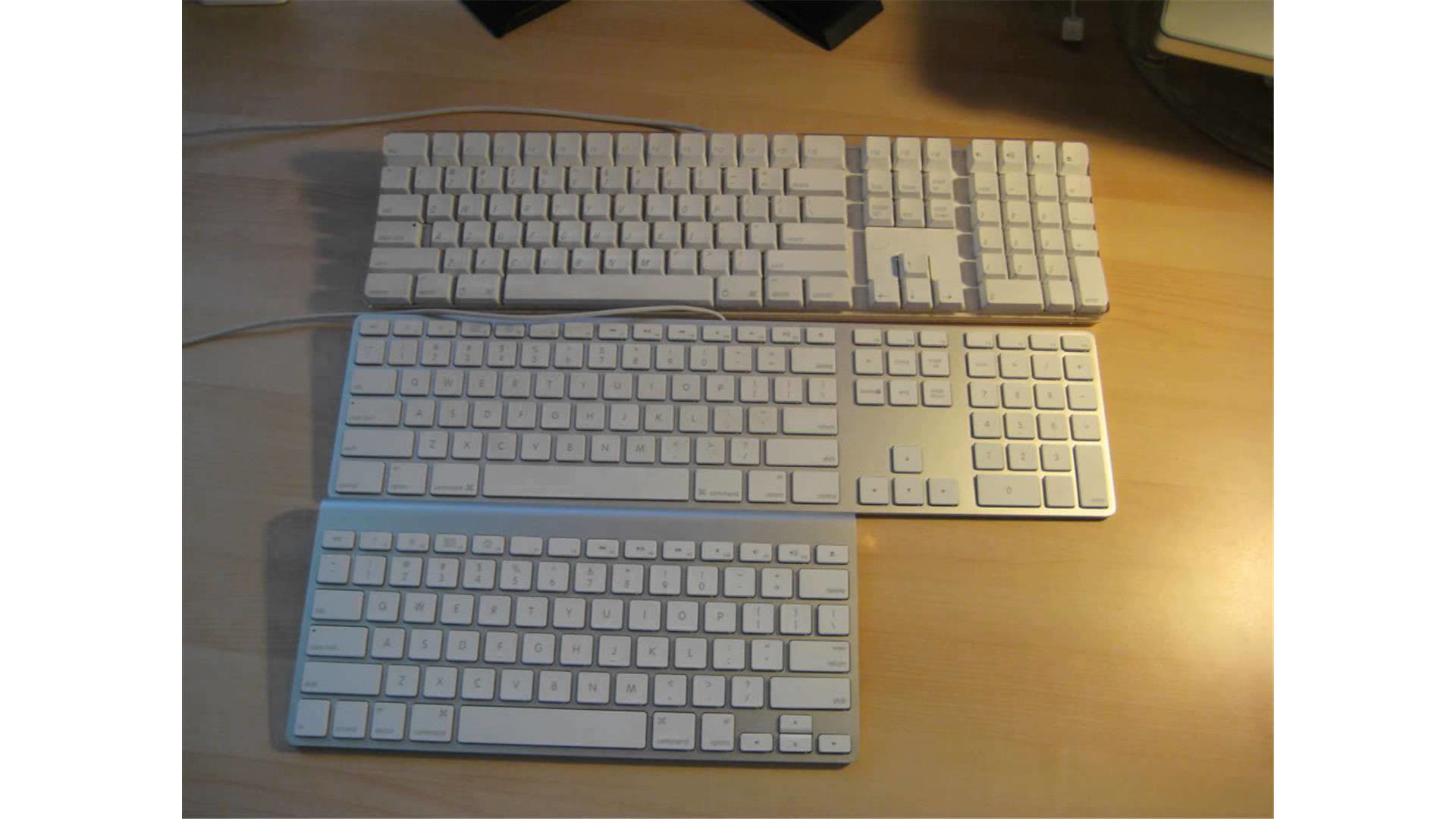The photograph features three white keyboards placed in a row, one above the other, on a light brown or beige tabletop. The image, taken on a shiny surface, is darkly lit with white reflections visible in the lower right corner. 

Starting from the bottom, the smallest keyboard lacks the number pad on the right side, making it shorter than the other two. This keyboard has low-set keys and a distinctive light blue horizontal line at its top. 

The middle keyboard is longer, featuring a number pad on the right side. It has low-set keys similar to the bottom one and includes a cord. This keyboard also has a white key layout against a light gray background.

The top keyboard is the largest, equipped with a number pad and a cord, like the middle one. However, it stands out with its high, cube-shaped keys, giving it an older, more mechanical design. 

In the top right corner of the image, there are cutout portions of black objects, adding a contrasting detail to the scene. The overall image captures the similarity yet distinct differences among the three keyboards, highlighting their design and functional variations.